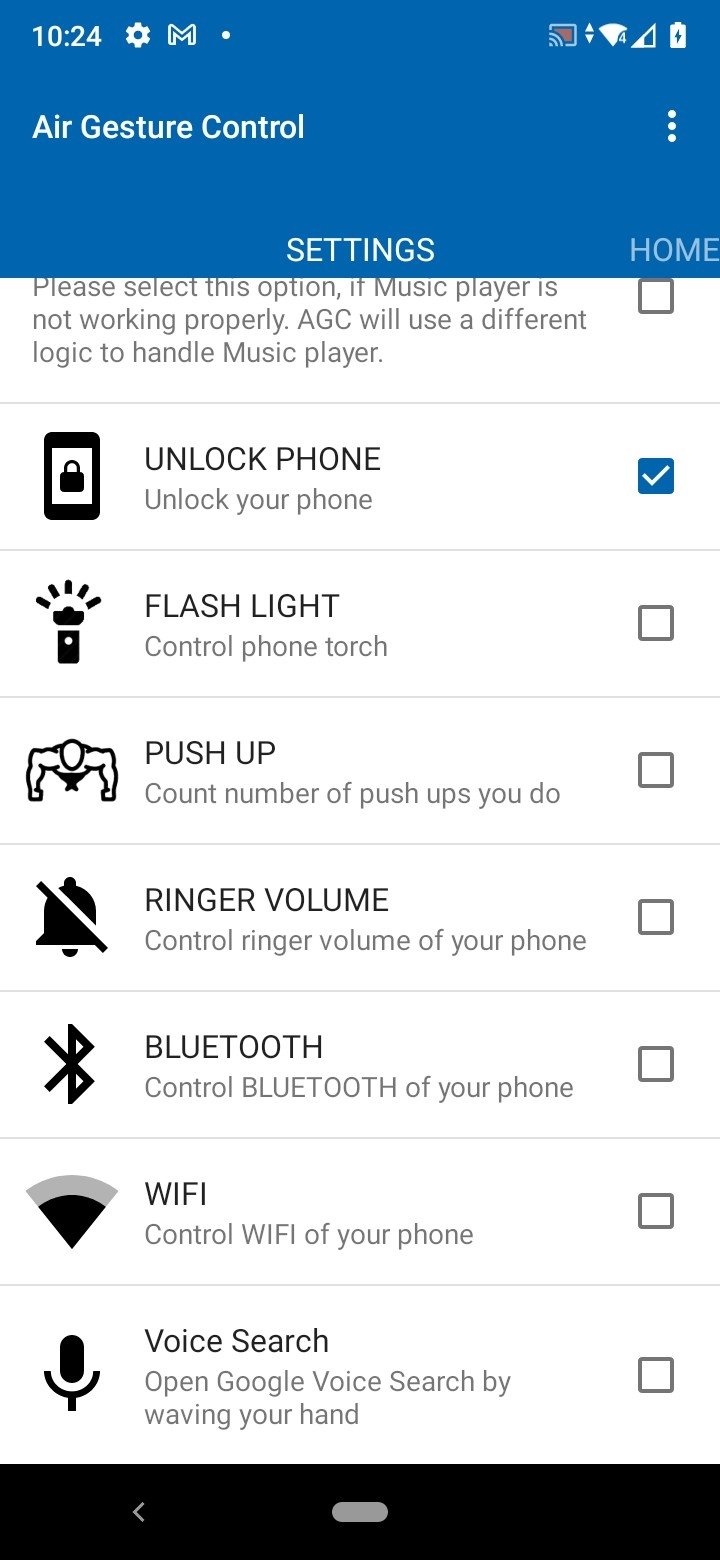This screen capture displays a cell phone's air gesture settings interface, providing a detailed overview of the current network connectivity and various setting options.

**Top Edge Status Bar:**
- **Top Right Corner:**
  - **Charging Indicator:** The phone is currently charging.
  - **Network Connectivity:** Two connections to cell towers with full Wi-Fi connectivity.
  - **Data Transfer Icon:** An icon showing an upward and downward arrow, indicating data transfer activity.
  - **Chromecast Active:** An icon indicating that Chromecast is activated.
  
- **Top Left Corner:**
  - **Time Display:** "10:24" with a gear icon representing settings and a Gmail logo followed by a dot.

**Main Screen:**
- **Background:** A blue backdrop with the title "Air Gesture Control" prominently displayed in the center.

**Overlay Elements:**
- **Buttons and Navigation:**
  - To the right side of the screen, slightly grayed out, "Home" is visible.

**Detailed Settings Menu:**
- A series of icons accompanied by text descriptions and checkmarks:
  - **Unlock Phone:** An icon of a cell phone with a lock, text "Unlock your phone" accompanied by a blue checkmark.
  - **Flashlight:** An icon of a flashlight, text "Control your phone torch" with no checkmark.
  - **Push-Up Count:** An illustration of a person doing a push-up, text "Count the number of push-ups you can do" with no checkmark.
  - **Ringer Volume:** An icon of a bell with a line through it, text "Control ringer volume of your phone" with no checkmark.
  - **Bluetooth:** The Bluetooth logo, text "Control Bluetooth settings of your phone" with no checkmark.
  - **Wi-Fi:** The Wi-Fi logo, text "Control Wi-Fi settings of your phone" with no checkmark.
  - **Voice Search:** A microphone icon, text "Open Google voice search by waving your hand" with no checkmark.

This detailed caption provides a comprehensive understanding of the cell phone's air gesture settings screen, highlighting both network status and the available gesture control options.